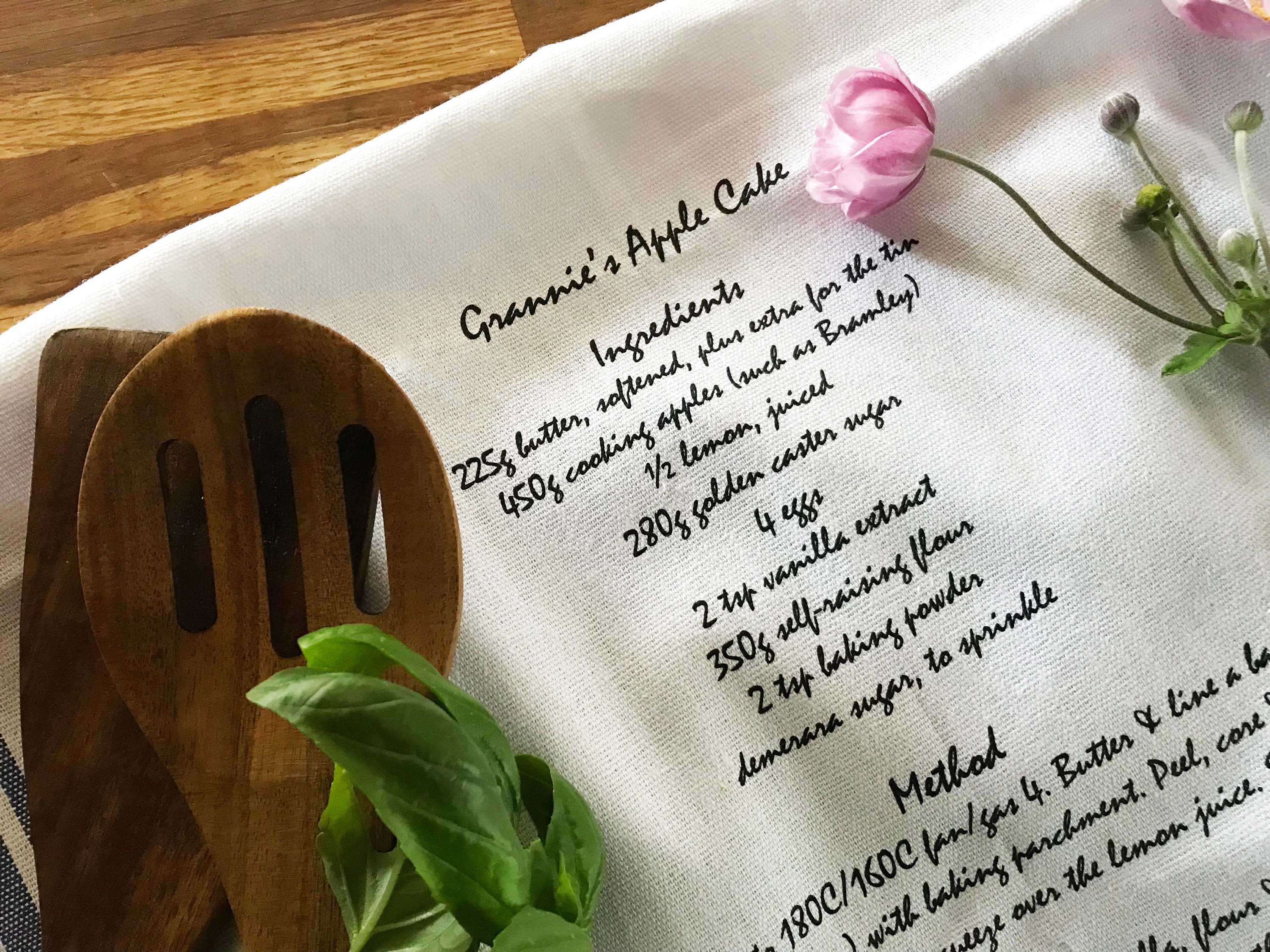The image depicts a professionally arranged white cloth on a brown wooden table. The cloth features a detailed, black cursive recipe titled "Granny's Apple Cake." The recipe includes a list of ingredients such as butter, 450 grams of cooking apples like Bramley, 280 grams of golden caster sugar, four eggs, two tablespoons of vanilla extract, among other components. Although the full methodology is provided, it is partially cut off at the bottom right corner of the image.

The cloth is set at a 45-degree angle from the top left to the bottom right of the frame. On the left side, there is a wooden spoon and a wooden spatula, accompanied by a piece of green leaf material. On the right side, a pink rose in bloom along with four or five unopened rose buds decorate the scene, adding a touch of elegance to the rustic setup. The arrangement accentuates the charm and homeliness of Granny’s Apple Cake recipe.